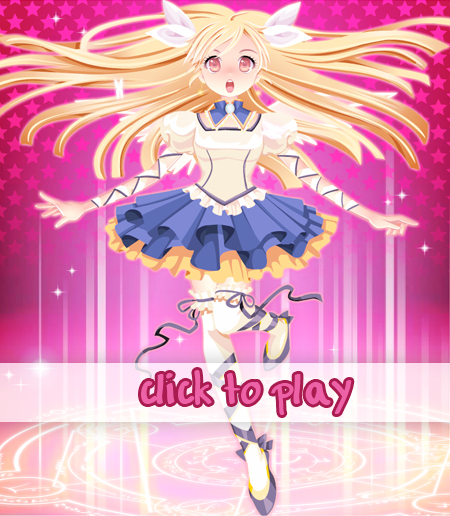This image portrays an animated female character, likely from a video game or anime. She is striking a graceful ballerina pose, standing on the tiptoe of her right foot while her left leg is bent and lifted. Her large eyes, which appear to be light brown or possibly pink, are wide open and convey a sense of surprise. Her mouth is also open.

The character has long, flowing blonde hair, with strands that fly out from each side of her head. She is adorned with peculiar white, leaf-shaped objects on her head that resemble ears, giving her an otherworldly appearance. Her dress is blue and white with two rows of frills: a top row of blue and a bottom row of light brown or gold. She completes the outfit with white stockings and black ballet slippers, although the slippers on her feet appear to be coming untied.

The background is a blend of purple and pink hues, filled with numerous small stars, especially concentrated around her head. Towards the bottom, there are stripes and lights that give the impression of a stage, supporting the idea that the setting might be a ballerina studio within a video game. The phrase "CLICK TO PLAY" is prominently displayed in pink or purple text within a white rectangular background, positioned near her legs. Overall, the image combines elements of fantasy and performance art in a visually striking way.